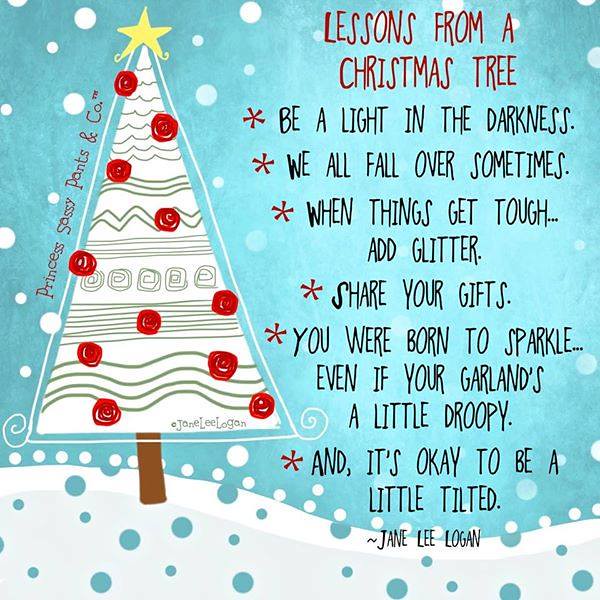The graphic design image showcases "Lessons from a Christmas Tree" prominently in red font at the top right. The background is blue and dotted to simulate falling snow, with a wavy white portion at the bottom where the falling dots transition to blue. On the left side, there's an artist's rendition of a pine tree: a white triangle adorned with green sketch marks for garlands and tinsel, alongside red squiggles representing ornaments. Near the base of the tree, in red text, it says "Princess Sassy Pants and Co."

The right side features a list in black font with red asterisks. The lessons listed are: "Be a light in the darkness," "We all fall over sometimes," "When things get tough, add glitter," "Share your gifts," "You were born to sparkle," "Even if your garland's a little droopy," and "It's okay to be a little tilted." At the bottom, this compilation of affirmations is attributed to Jane Lee Logan.